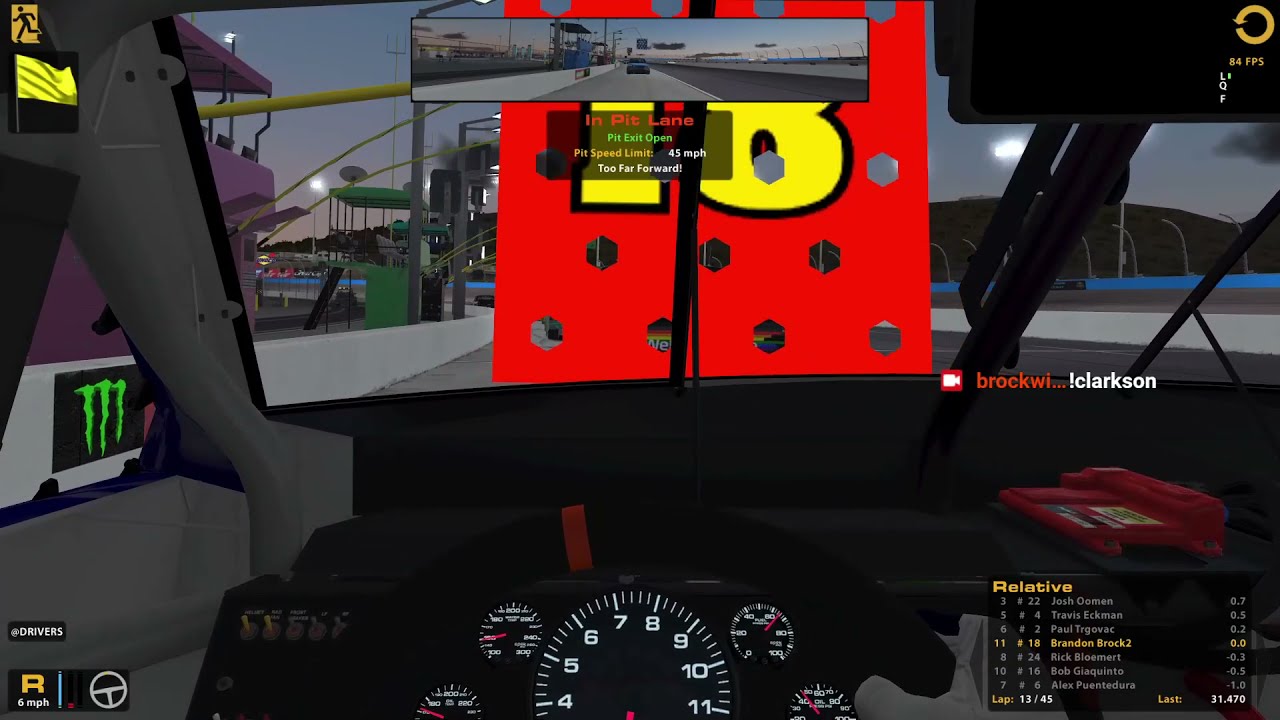The image depicts a screenshot from a racing video game, presented in a first-person perspective from the driver's seat. Dominating the center view is a bright orange block with holes, partially obscuring the windshield and displaying the yellow number "18." Above the block, red text reads "In pit lane," and green text announces "Pit exit open." Just visible through the windshield are elements of a racetrack, suggesting the car is either stationary or moving slowly within the pit area.

In the top middle of the screen, there's a small inset image displaying an exterior view of the vehicle on a roadway. To the right, red text lists "Brock W.I." and below it "Clarkson!" with additional data, possibly names and ranks, that are too small to discern clearly. The upper right corner features a circular symbol with an arrow.

On the lower left, a small steering wheel icon is accompanied by the letter "R" and the speed "6 mph," underlined by the word "drivers." Another icon of a running man, seemingly exiting through a door, sits in the upper left corner. Amidst the visual clutter, a partially legible area suggests a pit speed limit set at 45 mph. The details combine to convey the immersive experience of being at the wheel within a vibrant and detailed racing simulation.